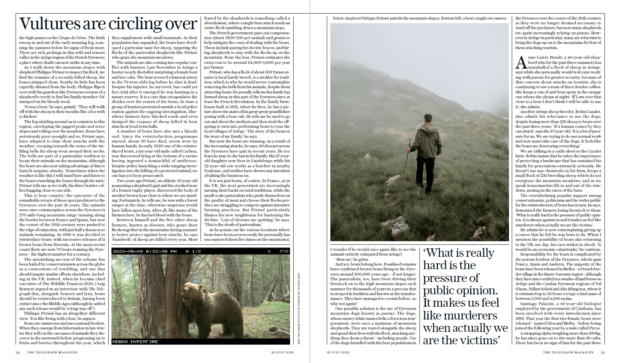This screenshot captures the first two pages of a publication. On the left side, the first page features the prominent headline "Vultures Are Circling Over" in large black text located in the upper left corner. The text beneath is divided into three columns, but the font size is too small to read further details. In the lower right corner, there is a vivid photograph of a brown bear in the woods. The bear is depicted with its head leaning against a tree trunk to the left of its body. Our view is of the bear's right side as it faces west, standing on lush green grass amidst a densely forested background.

On the right side, the second page includes a striking image of a man standing on a mountain with his back to the viewer, holding a walking stick. Alongside this picture, there is an evocative quote: "What is really hard is the pressure of public opinion. It makes us feel like murderers when actually we are the victims." The images and texts together present a compelling narrative within the publication, blending stark natural imagery with poignant reflections on public perception.